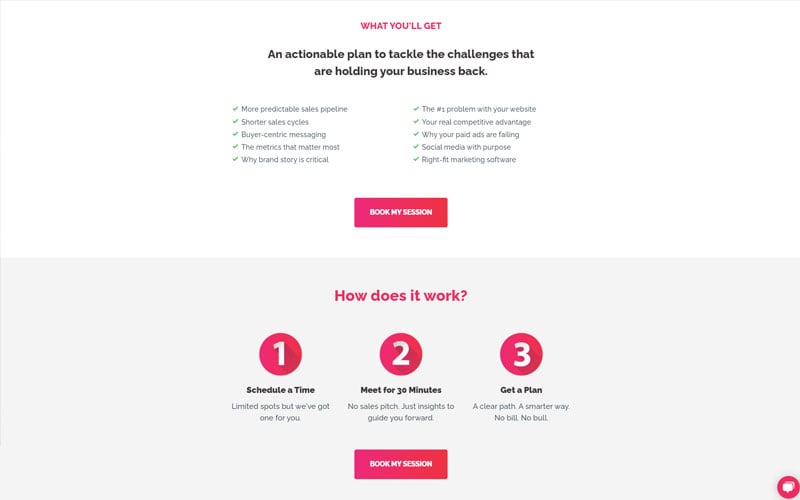**Detailed Description:**

The image is a screenshot of a business management service interface, characterized by a predominantly white background at the top and a light gray background occupying the bottom third of the image. 

At the top of the image, there's a headline in red text stating, "What you'll get." Directly below this, a bold black text highlights the primary offering: "An actionable plan to tackle the challenges that are holding your business back." 

Following the main description, a two-column list enumerates five key benefits, each item accompanied by a small green checkmark:
- Column one lists:
  1. More predictable sales pipeline
  2. Shorter sales cycles
  3. Buyer-centric messaging
  4. The metrics that matter most
  5. Why brand story is critical

Below this list, a prominent red rectangle with white text reads, "Book my session."

Transitioning to the bottom section with the light gray background, a heading in red text asks, "How does it work?" Underneath this, three red circles, each containing white numerical text (1, 2, 3), describe a simplified process:
1. Schedule a time
2. Meet for 30 minutes
3. Get a plan

Each step includes a brief text description. At the bottom, another red rectangle with white text reiterates, "Book my session."

In the bottom right corner, there is a small red circle with a messaging icon, likely indicating an option to leave a message or engage with a chatbot.